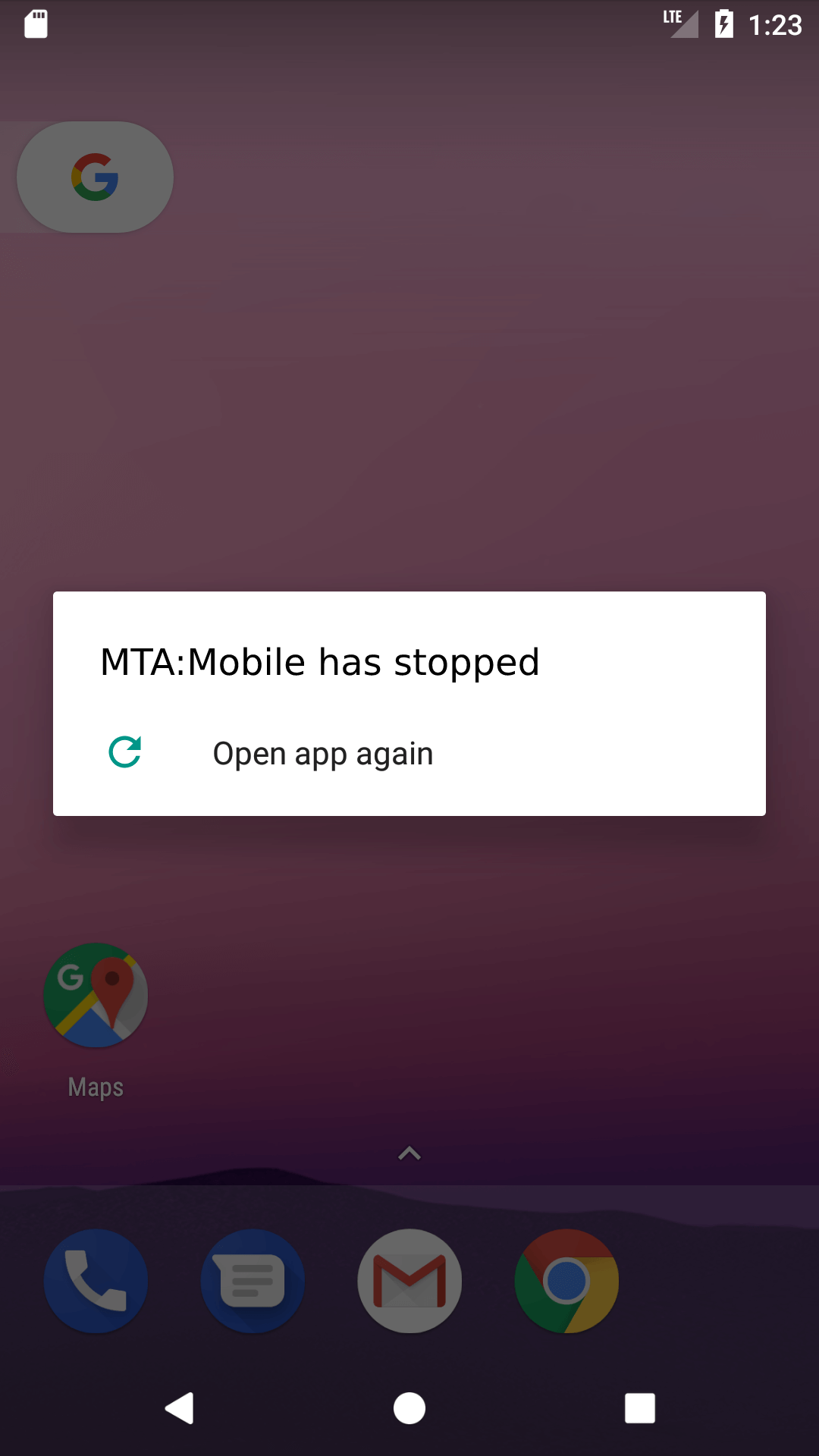The image is a screenshot of a smartphone screen, with a purplish-pink background. In the very top left corner, there's a small white save icon, followed by "LTE" to the right. Adjacent to it, there's a battery symbol with "123" next to it. Below the save icon is the Google logo, characterized by a white oval containing a multicolored "G."

The central part of the image features a notification box with a white background. The box displays an error message: "MTA Mobile has stopped," accompanied by a green clickable arrow labeled "Open app again." Below this, the Google Maps icon is visible, showcasing its characteristic green, yellow, red, blue, white, and gray colors.

The bottom section of the phone screen displays four prominent app icons: a blue and white phone symbol, a blue and white messaging symbol, a red and white Gmail symbol, and a colorful Google Home icon with red, yellow, green, and blue hues.

At the very bottom of the screen are navigation buttons: a white rectangle, a white circle, and a white square, lined up horizontally.